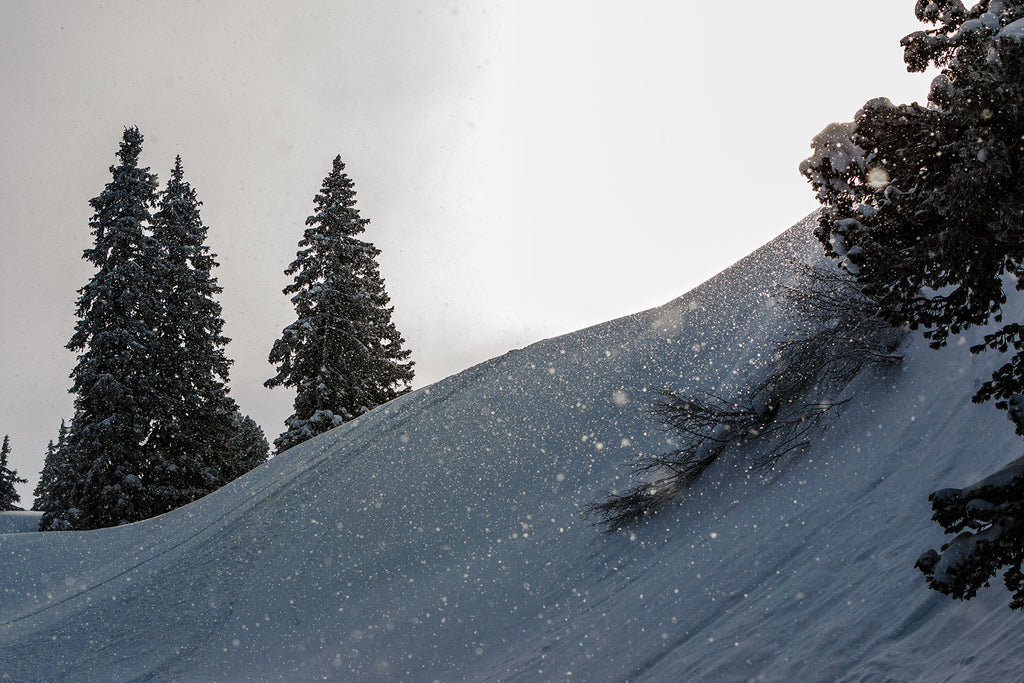The image captures a serene winter scene dominated by snowy slopes and pine trees. The landscape features a snow-covered hill that ascends diagonally from the lower left to the upper right. The upper left corner of the sky is a deep gray, transitioning to a lighter gray towards the top right where faint sunlight filters through. Snowflakes cascade gently, resembling fine salt grains. On the left side, fully visible pine trees stand tall, while the right side reveals partial views of tree branches, some fallen and poised as if they might slide down the slope. The snow in the bottom right corner appears disturbed, with shallow indentations suggesting recent activity, possibly ski marks or footprints. This picturesque scene beautifully blends the tranquil snowfall with the rugged terrain and evergreens.